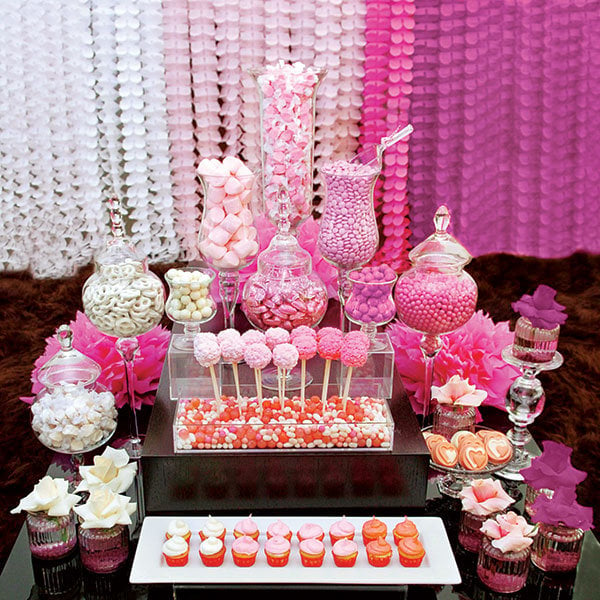This photograph showcases an elaborate party dessert table adorned with a myriad of sweets and decorated in a harmonious palette of pink, purple, and white. At the forefront, a small tray of cupcakes garnished with white, pink, and orangey-pink frosting sits, each with a red cupcake holder. Flanking these cupcakes are charming jars filled with white, pink, and purple flowers placed atop pink beads. 

In the center, there are two rows of lollipops - pink ones in the front and darker pink ones in the back - arranged in a tray filled with various red, pink, and white sweets. Surrounding these lollipops are five glass jars of candies, organized by color. On the left, jars contain white pretzels and lighter treats, while those on the right contain reddish-pink and purple candies. The middle jar, the tallest among them, is packed with pink-wrapped lollies, and another jar sports a scoop for easy serving. Further details include glass containers brimmed with marshmallows, yogurt pretzels, hard candy, and jelly beans.

Enhancing the table’s festive atmosphere, a large glass vase centrally located contains delicate flower petals. In the backdrop, ornamental drapes transition in color from white on the left to darker pinks, finishing with purples on the right, adding an elegant touch to the setting. The combination of vibrant flowers, an assortment of treats, and meticulously coordinated decorations highlights the celebratory ambiance captured in this photograph.